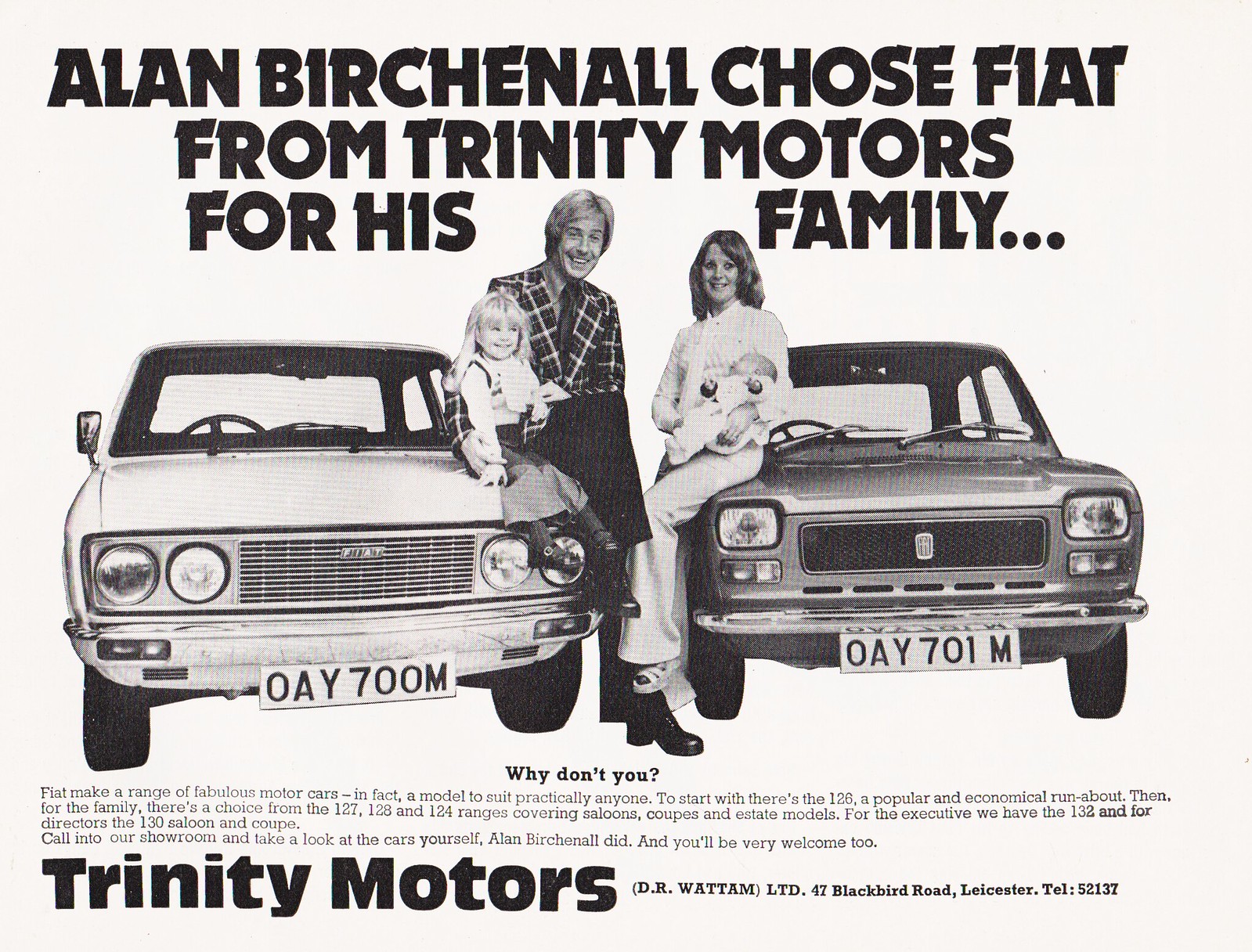This black and white magazine advertisement for Trinity Motors showcases Alan Bertchanal and his family's choice of Fiat vehicles. At the top of the ad, bold, uppercase text proclaims, "ALAN BERTCHANAL CHOSE FIAT FROM TRINITY MOTORS FOR HIS FAMILY." The image features two cars: on the left, a larger white Fiat with a license plate reading 0AY700M, leaned on by a blonde man in a plaid sports coat, tie, and button-down shirt. He holds a small, blonde girl dressed in a white shirt and skirt, who sits on the car's hood. On the right, there's a smaller, lighter-shaded Fiat with the license plate 0AY701M. A woman with shoulder-length hair, dressed entirely in white pants and a shirt, leans on this car while holding a baby. The bottom of the ad asks, "Why don't you?" followed by a descriptive paragraph highlighting the versatility and range of Fiat models, further emphasizing their appeal to different customer needs. The ad concludes with the bold "TRINITY MOTORS" logo and smaller text providing the dealer's address and contact number: D.R. Wadham Limited, 47 Blackbird Road, Leicester, Telephone 52137.